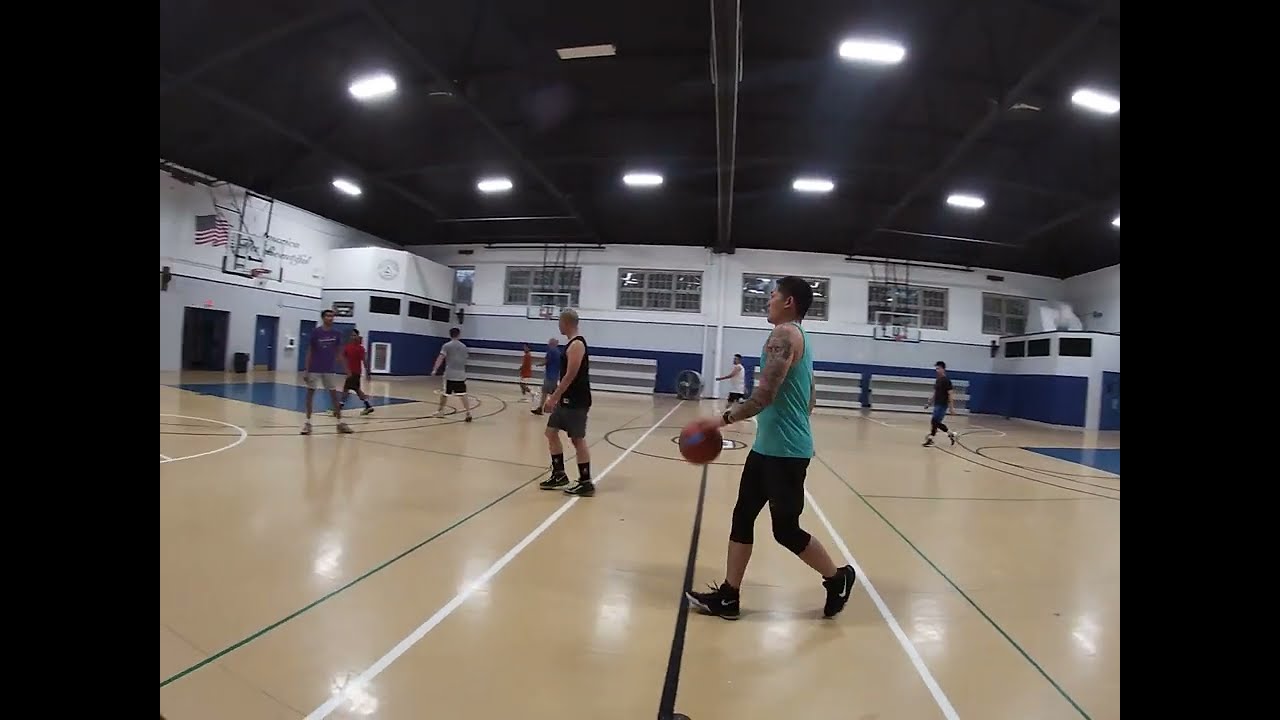This photograph captures a dynamic scene of a basketball game taking place in an indoor gymnasium at night. The gym features a beige basketball court marked with white, blue, and forest green lines. The bright indoor lights illuminate the space, revealing multiple tall windows that look out into the dark night and a black ceiling. An American flag hangs on the upper left part of the wall behind a basketball hoop, with collapsed bleachers visible in the background.

In the center of the image, a man with dark hair and a tattooed left arm is dribbling a basketball as he moves from right to left. He wears a sleeveless mint green tank top, black capri leggings, and black Nike sneakers with a white swoosh logo. A black watch adorns his wrist. Surrounding him, eight other players are positioned across the court. They are dressed in various athletic outfits, including tank tops, shorts, and sneakers, in colors such as teal, gray, purple, red, and dark blue. The overall atmosphere is vibrant and competitive, capturing a moment of intense focus and movement in the game.